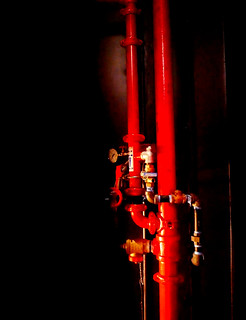A striking image showcases a fire engine red pipe, set against a stark black background. The pipe, rising vertically from the bottom, branches out into a secondary pipe about one-third up its length. Adorned with intricate golden accoutrements and attachments, the pipe exudes a steampunk aesthetic pushed to the extreme. The top section of the pipe appears slightly narrower than the base, lending an unusually distorted and somewhat surreal quality to its form. The overall visual impression suggests the image could be AI-generated, due to its slight fuzziness and unconventional proportions. This steampunk-inspired creation captivates with its vivid colors and elaborate detailing.